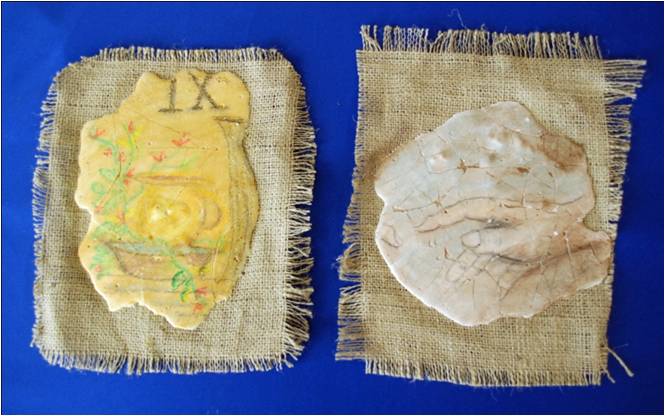In this overhead photograph, two flat stones with detailed carvings and paintings are showcased against a bright blue tabletop. Each stone lies on a piece of burlap sackcloth. The stone on the left is irregularly shaped, predominantly yellow, with the Roman numeral "IX" inscribed on the top. This stone features a painted scene of a flower pot containing red and yellow flowers with green stems, accompanied by a small bowl of water in front. The stone on the right is white and depicts a faint yet discernible drawing of a hand reaching towards another hand, reminiscent of the iconic image of God's hand reaching out from the heavens. The delicate details and the contrast of the stones against the vivid blue background and rustic burlap create a striking visual.